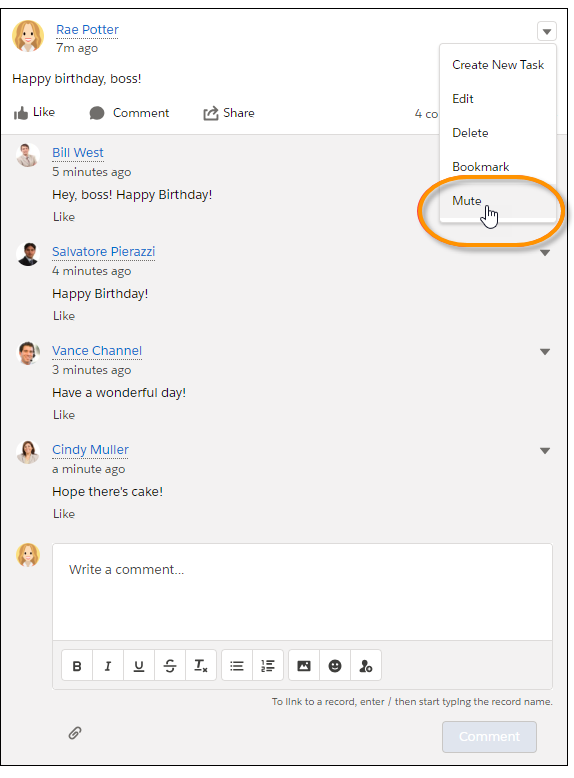This image is a cropped screenshot of a post from a company message board. In the upper left corner, a circular profile picture of the user is displayed. To the right of the profile picture, the user's name, Ray Potter, is highlighted in blue and underlined with dashes, indicating it is a clickable link. Directly below her name, it is mentioned that the post was made 7 minutes ago. Ray's comment reads, "Happy birthday, boss."

Below the comment, there are three interactive buttons: a like button, a comment button, and a share button. In the top right corner of Ray's post, a downward-pointing arrow has been selected, revealing a vertical menu with options such as "Create New Task," "Edit," "Delete," "Bookmark," and "Mute." The word "Mute" is encircled in red, emphasizing the option to mute the conversation.

The post has accumulated four comments, though only the number is visible as the comments are not displayed in the screenshot. The person who authored the post appears to be the one who took the screenshot. At the bottom of the post, aligned to the left, Ray's profile picture reappears next to a large white text box labeled "Write a comment." Beneath this text box, there is a horizontal array of formatting options, including bold, italic, underlined text, text size adjustments, emojis, and an option to insert a photo.